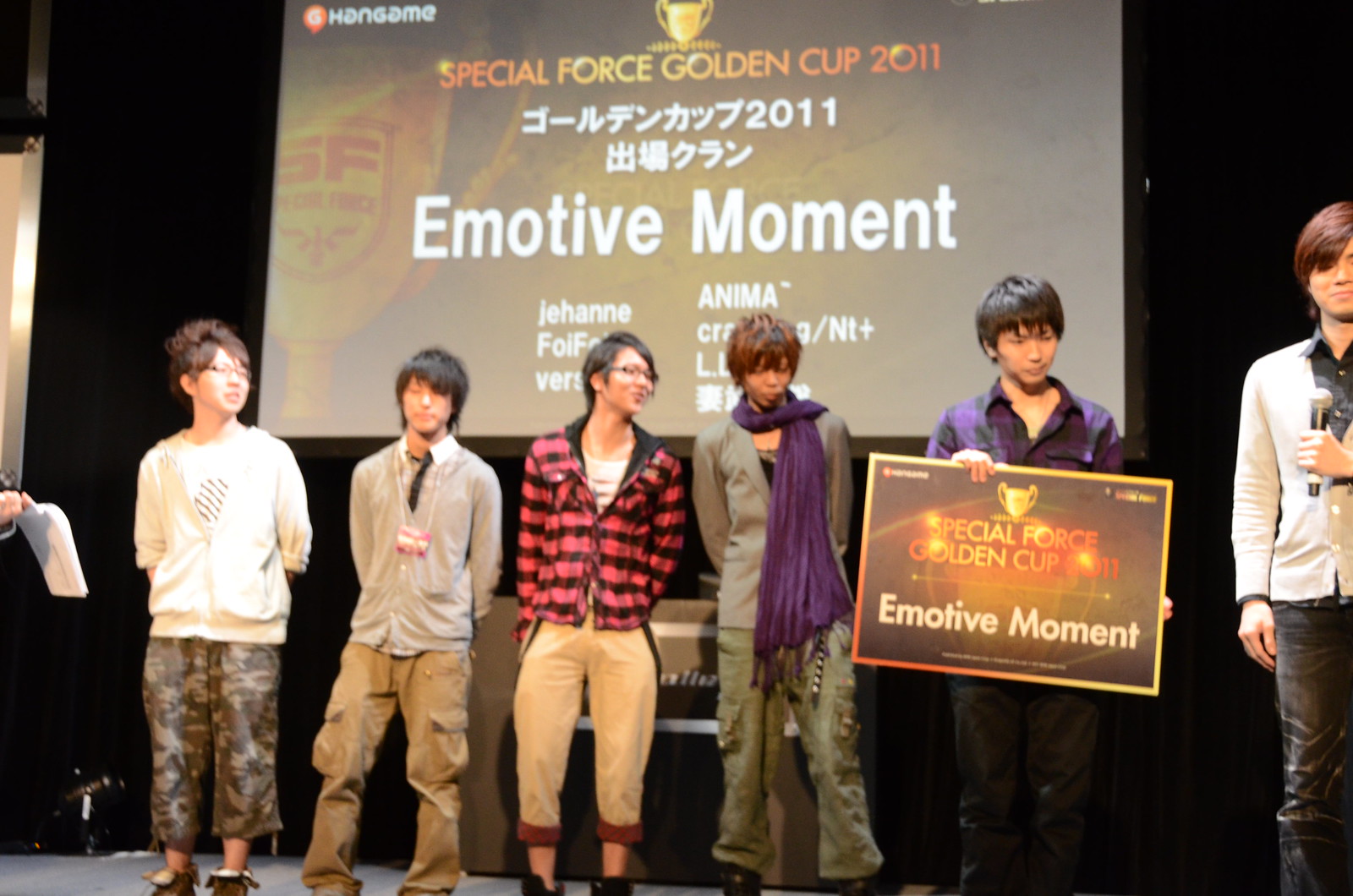Six young men are standing on a stage with a large projector screen behind them. The screen, decorated with a big banner, prominently reads "Special Force Golden Cup 2011" and "emotive moment" in white text, accompanied by various other texts in Japanese. Starting from the far right, there's an Asian man with brown hair combed over his left eye, wearing a white shirt with a black collar, denim-colored pants, and holding a microphone in front of his chest, with the other hand by his side.

Next to him is a young boy with black hair covering his forehead, sporting a purple and black plaid shirt. He holds a poster featuring a gold cup in the center, outlined in gold, with the words "Special Force Golden Cup" and "emotive moment" in white text against an orange, shiny background.

Next is a girl with messy brown and black hair, wearing green pants, a gray jacket, and a distinctive pink scarf that extends down between her legs. Beside her stands a person in a red and black plaid jacket over a white shirt, wearing black glasses and khaki pants with brown stripes around the ankles, looking to the right.

Following them is a young man with messy black hair, donning a gray button-up shirt with a necktie tucked inside, and khaki pants. Lastly, there's a young lady with her hair standing up in the middle, dressed in a white sweatshirt, camouflaged pants, and glasses, facing to her right with her arms tucked behind her back.

All these individuals appear to be Asian and dressed in varying casual and semi-casual attire, creating an ensemble reminiscent of a boy band. Behind them, partially obscured, additional text reveals "J-e-h-a-n-n-e" and "A-n-i-m-a," with a hand and some white paper visible at the far left edge of the image.